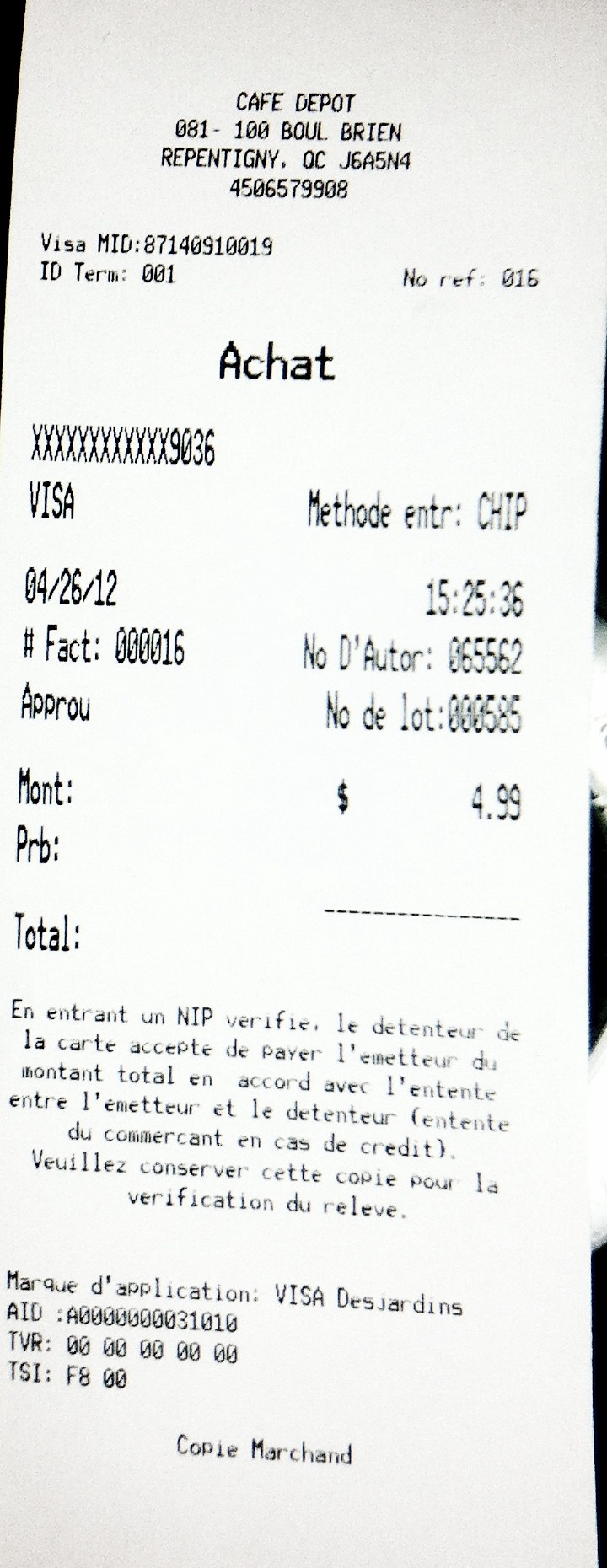This image is a close-up photograph of an old-fashioned register receipt printed on register paper. The print is tiny but legible in some parts. At the very top, it features the header "Café de Port," followed by the café's address, which is partially obscured. The receipt indicates that the payment method was Visa card, marked clearly both at the center and the left side of the receipt. 

Below the address, the foreign word "ACHAT" appears, hinting at a non-English language, likely French, meaning "purchase." On the right side, the term "Method" followed by "Chip" is visible, suggesting that the payment was made using a chip reader. 

The transaction date is noted as April 26, 2012 (formatted as 04-26-12), with a timestamp of 15:25:36, indicating the precise time of the purchase. The total amount for the transaction is prominently displayed at the bottom as $4.99.